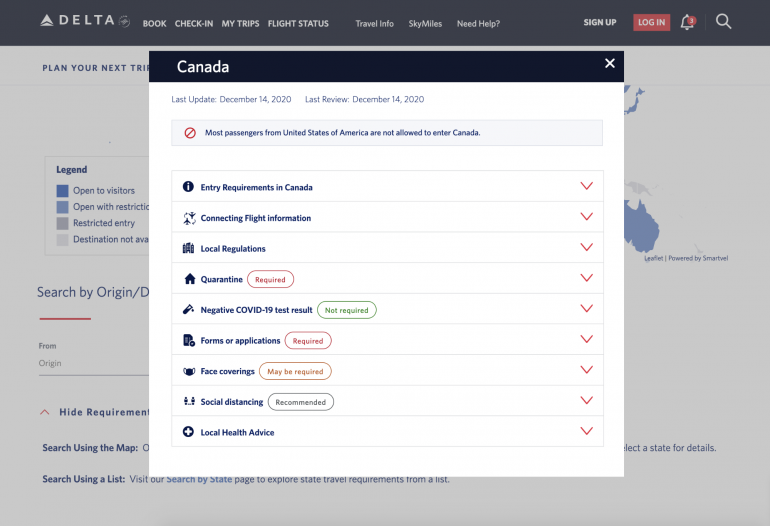The image is a screenshot from the Delta website, characterized by a distinct, sleek design. At the top, a black navigation bar spans the width of the image, featuring the Delta logo and the word "Delta" in white text on the upper left. Adjacent to this, a series of tabs are displayed across the bar: ‘Book,’ ‘Check-in,’ ‘My Trips,’ ‘Flight Status,’ ‘Travel Info,’ ‘SkyMiles,’ ‘Need Help,’ ‘Sign Up,’ ‘Login,’ and a notification bell with a red indicator showing three pending notifications, followed by a search icon on the far right.

The primary background of the image is white, but it's mostly obscured by a pop-up screen. This pop-up screen also has a black header bar which displays the word "Canada" on the upper left, accompanied by a warning or stop symbol. Beneath this bar, a critical message is prominently displayed: "Most passengers from the United States of America are not allowed to enter Canada." 

Following this alert, there's a detailed list of information pertinent to travelers, encompassing entry requirements in Canada, connecting flight information, local regulations, quarantine protocols, the necessity of negative COVID-19 test results, forms or applications, face covering mandates, social distancing guidelines, and local health advice.